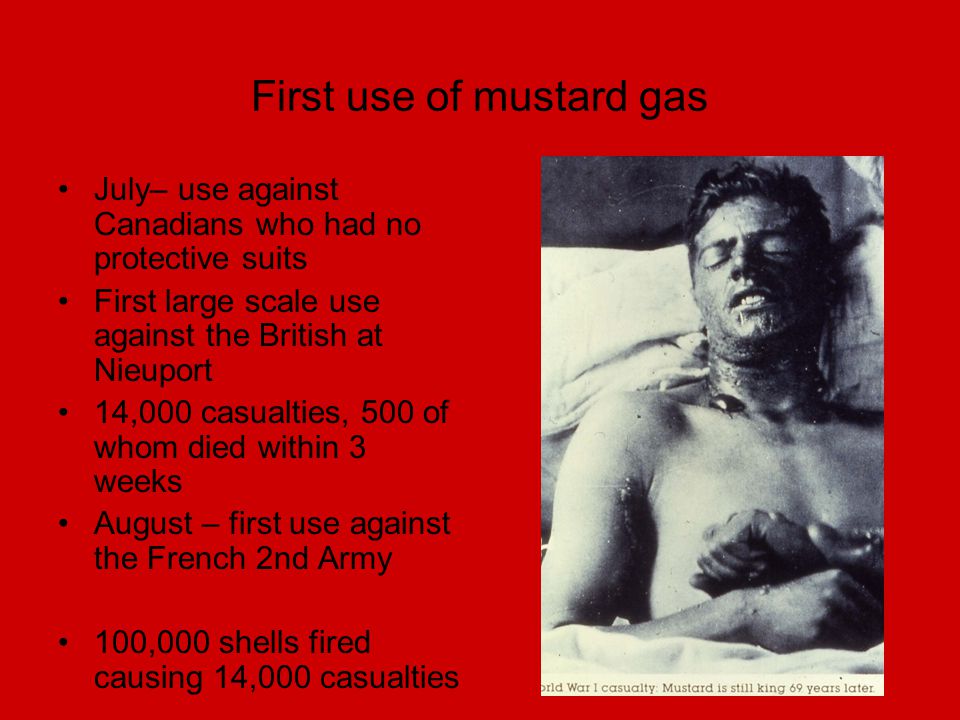The image, featuring a dramatic solid red background with stark black text, presents detailed information on the first use of mustard gas. At the top center, the title reads "First Use of Mustard Gas" in bold black letters. On the left side are five bullet points providing chronological details of its deployment: "July - Use against Canadians who had no protective suits," "First large-scale use against the British at Newport," "14,000 casualties, 500 of whom died within three weeks," "August - First use against the French Second Army," and "100,000 shells fired causing 14,000 casualties."

On the right side, there's a haunting black-and-white image of a man in apparent agony. He is shirtless, lying against what seems to be a pillow, with his eyes closed and mouth open, possibly a World War I casualty suffering from mustard gas effects. His hands appear to be clasped or shackled. Below this distressing photograph reads the caption: "World War I casualty, mustard is still king 69 years later." The image seems to be designed as a poster or presentation slide to vividly convey the harrowing impact of mustard gas during the war.